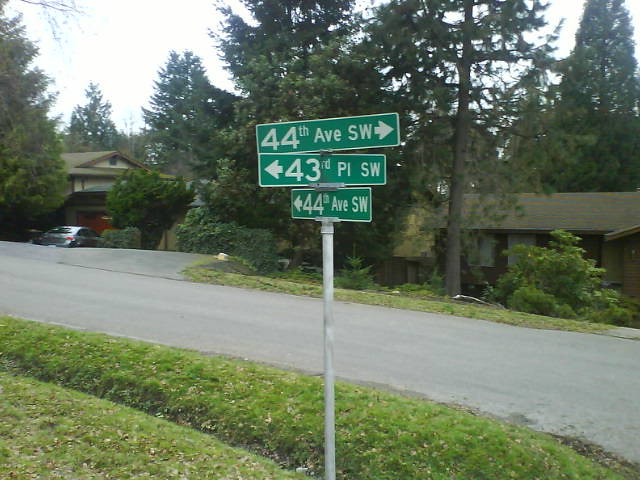The image captures a detailed street corner in a suburban residential neighborhood with elements suggesting it might be Seattle. A metal street signpost stands centrally, displaying three stacked directional signs. At the top, a white arrow points right with "44th Avenue SW." Below, another white arrow directs left to "43rd Place SW." The lowest sign again points left but more toward the back, indicating "44th Avenue SW." Surrounding the signpost are tall evergreen trees and leafy greenery typical of a woody area. In the background, two brown, low-slung ranch houses with asphalt shingled roofs are visible, nestled among the trees and shrubs. One of the houses, on the left, has a distinctive red garage door with a Porsche Carrera parked in front. The neighborhood appears peaceful with a road devoid of lane markings, flanked by grass and a ditch on the left side of the viewer’s perspective, indicating a quiet, residential ambiance.